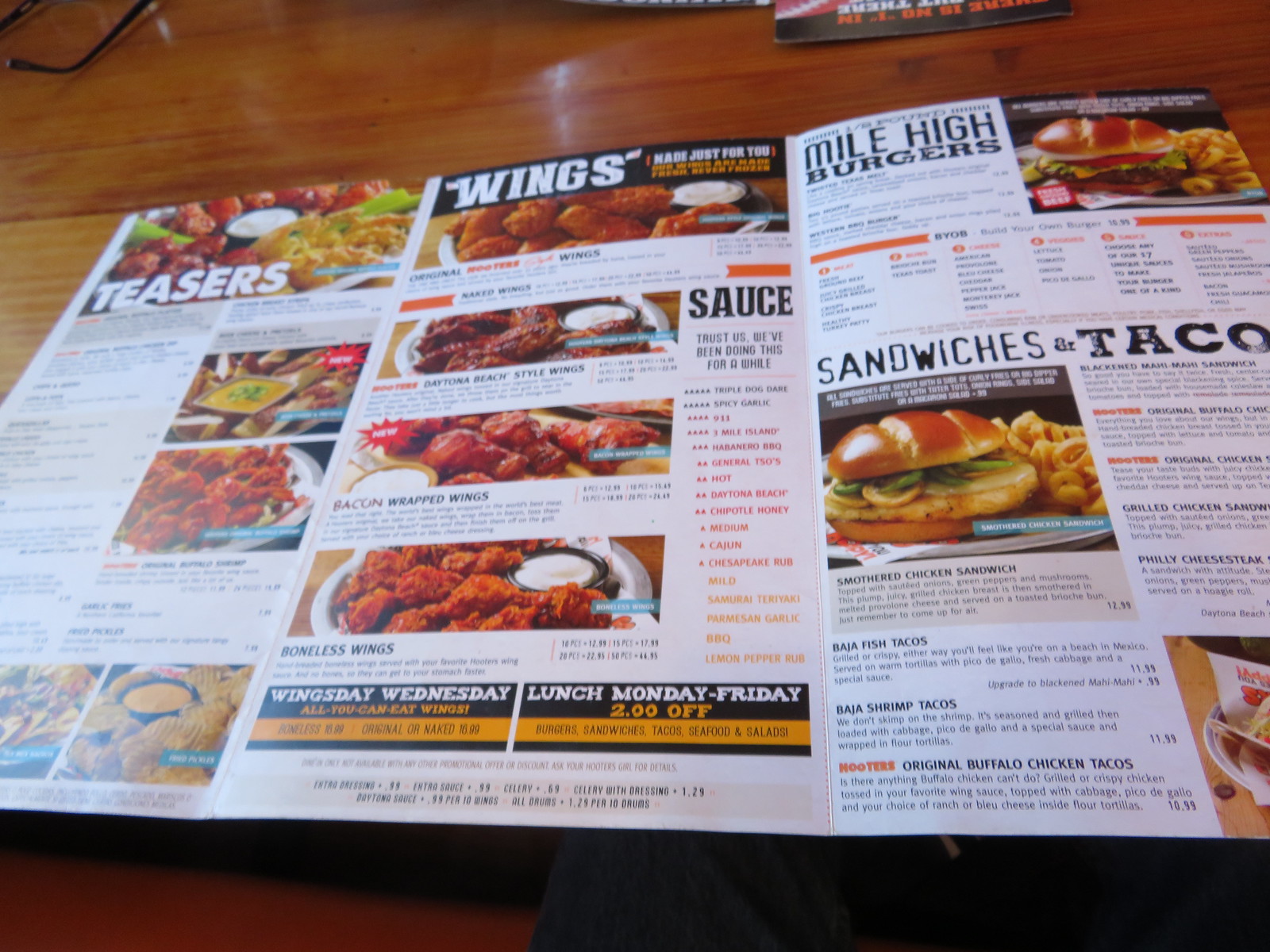In this large square image, we see an open, tri-fold menu laid out on a brown wooden table in a fast casual restaurant. The menu is prominently positioned in the center of the photograph, detailing a variety of food items. The left side of the menu features a section titled "Teasers" in large white letters, accompanied by a cluster of appetizing pictures in the upper left corner, showcasing various appetizers. Below this, another section highlights different styles of wings, including "Mixed Wings," "Daytona Beach-style Wings," and "Bacon-wrapped Wings," each with a respective rectangular photo and a brief, albeit unreadable, description in black text. 

The right side of the menu starts with a section named "Mile-high Burgers," adorned with a picture of a juicy burger to its right. Following this, the menu lists sections for "BYOB" (Build Your Own Burger), "Sandwiches," and "Tacos," each with enticing images and additional menu items. A delectable sandwich paired with curly fries is also featured in the middle part of the right side. Adding to the visual appeal, the menu includes various vibrant colors such as black, brown, orange, yellow, green, and red. The setting of this scene clearly indicates an indoor restaurant environment where additional objects like glasses and another closed menu are visible toward the upper left corner and top of the image, respectively. The menu also contains advertisements at the bottom for specials like "Wednesday Wing Day" and a "Lunch Special", enhancing the inviting and vibrant presentation of the overall dining offerings.